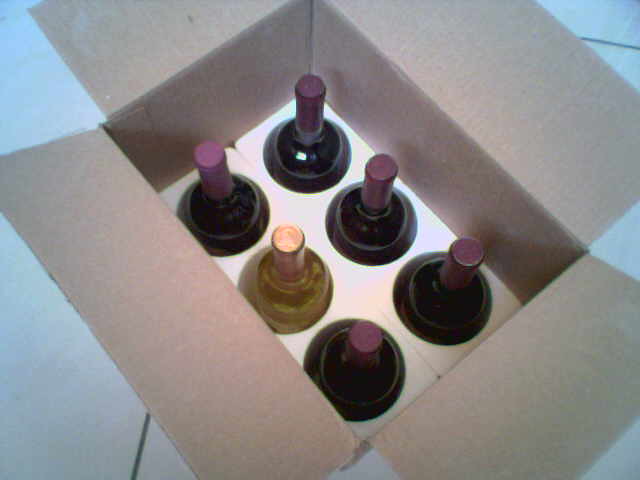The photograph depicts an open cardboard box placed on a floor with white square tiles and grayish grout. Inside the box is a white styrofoam insert with six cut-out holes arranged in a two-by-three configuration, securely holding six wine bottles. Five of the bottles, positioned in the top two rows and the bottom corners, appear to contain a very dark liquid, likely red wine, sealed with maroon or black foil coverings. The remaining bottle, located in the left center, contains a yellowish liquid indicative of white wine and is sealed with a yellow foil wrapper around the neck. Shadows of the bottles and reflections from a flash are visible on the styrofoam, enhancing the texture and depth of the image.